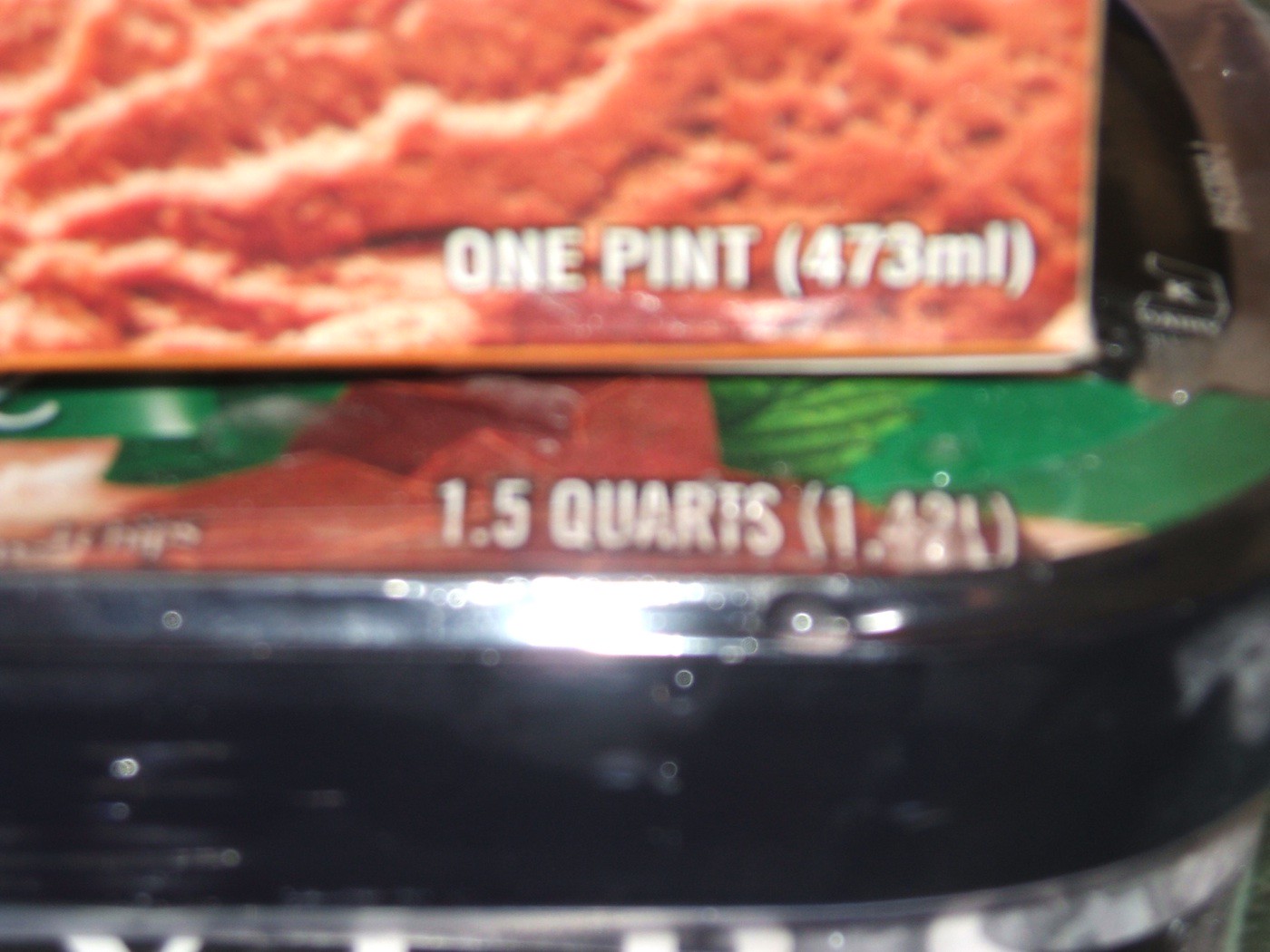This photograph, likely taken with a flash, depicts an extremely blurry close-up of two different kinds of food packaging on a shiny black surface, possibly metal, creating noticeable reflections. The upper portion of the image shows the bottom right of a rectangular box with a rough texture and brown coloring. In bold, white capital letters, it states "1 PINT" with "473 ML" in parentheses. Below this, partially obscured, another food packaging is visible, featuring a mix of green and red hues. This lower label, also in white capital letters, reads "1.5 QUARTS" with "1.42 L" in parentheses. The glare in the lower center and some green reflections on the black surface further obscure the image.